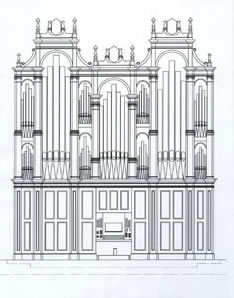This intricate black-and-white, computer-generated architectural drawing depicts the interior of a Renaissance-style cathedral, characterized by three towering sections, with the two outer towers slightly taller than the central one. The line work is exceptionally fine and precise, suggesting the use of a computer program to achieve such meticulous detail. The structure features a significant number of architectural points and decorative spires, adding to its ornate appearance. The tall outer towers each house five large pipe organs, reminiscent of elongated fingers, while the shorter middle section includes seven slightly higher organ pipes. At the base of these towers, speakers and an organ can be seen, positioned centrally beneath an elevated screen, hinting at a modernized, multi-functional use within this grand, historical-inspired design. The entire layout is rendered in stark black ink against a white background, highlighting the detailed geometric patterns and architectural pillars that define the building's majestic form.